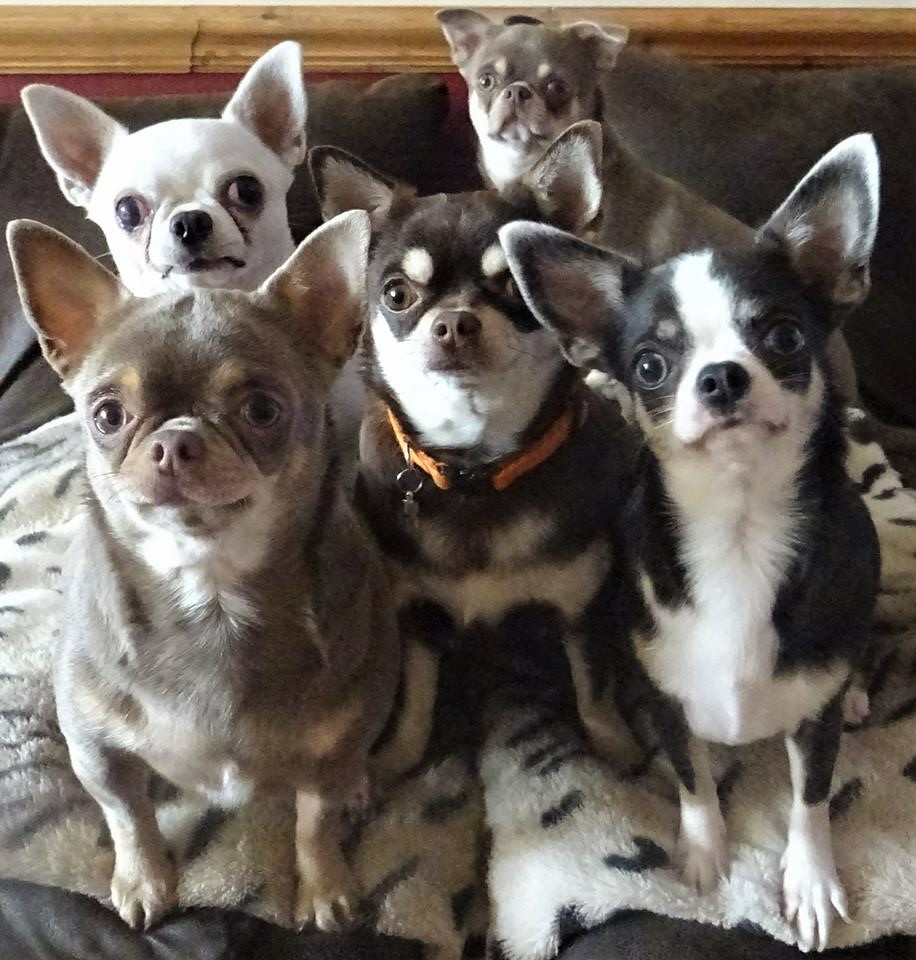This square-format color photograph captures an adorably engaging scene of five small dogs, all of the same breed—likely Shih Tzus—perched cozily on a soft, dark gray couch or bed adorned with a gray blanket featuring black and white striped patterns and accompanied by two gray pillows. Each dog captivates with its distinct coat: the dog on the front left is light gray with white patches, the one next to it flaunts a darker gray with white around the neck and face, enhanced by an orange collar. The centrally positioned dog showcases a charming mix of black and white with large, pink-tinged ears. Behind, one dog, predominantly gray with some white, faces sideways but turns its head to lock eyes with the camera. The last dog's head, primarily white with a black nose, peeks out from behind. All five dogs, with their grumpy yet endearing expressions, sharp nails, little legs, short necks, and pointy ears, are keenly staring at the viewer, creating a delightful and unified gaze towards the camera.